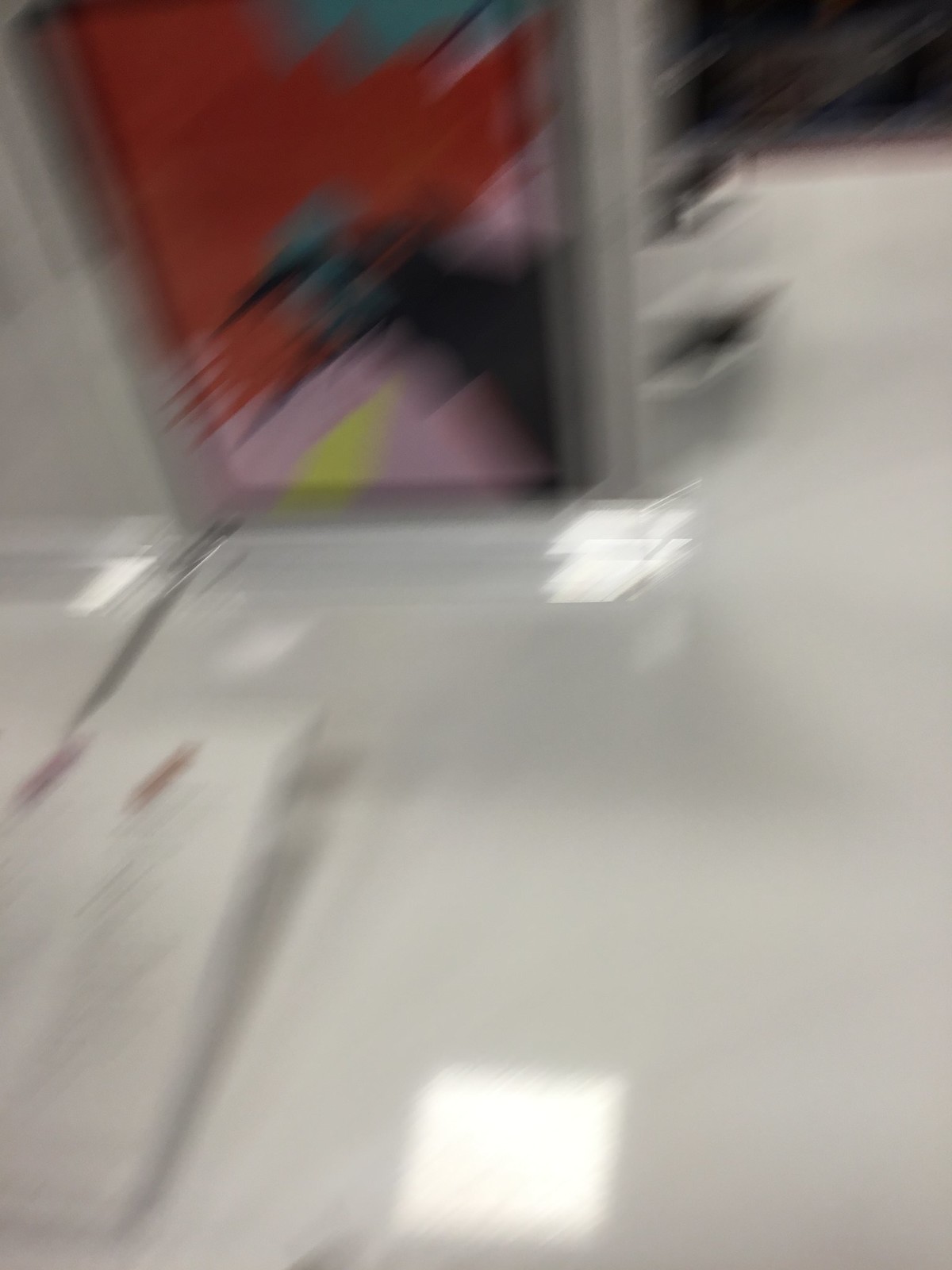This is a blurry, low-resolution color photograph in portrait format, depicting an indoor setting that appears to be either an airport or a mall. The motion during the image's capture moves from the top right to the bottom left, resulting in a clear directional blur. The floor is a very shiny, possibly white linoleum, reflecting the overhead lights, which create squares of glare on the surface. Along the wall, there is an artistic design featuring a mix of red, pink, yellow, and blue hues. In the top left-hand corner of the photo, there seems to be an advertisement or sign, characterized by blocks of color in red, pink, black, and blue, with hints of yellow. Additionally, there might be a piece of paper lying on the floor.